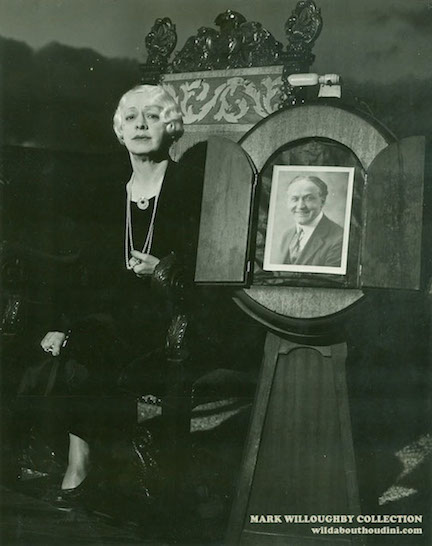This meticulously detailed black and white photograph showcases an older woman seated in a highly ornate wooden chair adorned with intricate filigree engravings and a gothic-style back that extends well above her head. She exudes a serious demeanor and is dressed in mid-20th century attire, featuring a low-cut black dress complemented by long, small pearl necklaces and black shoes. Her white hair, styled in a reminiscently 1920s-1930s finger wave, is beautifully curled. The woman holds onto one of her pearl necklaces with one hand. To her right stands an elaborate display, featuring a circular board atop a pylon, which contains a black and white photograph of a smiling man, identified as Harry Houdini. The display's base is noted to have small doors on the front. At the bottom right corner of the overall image, white text reads: "Mark Willoughby Collection, wildabouthoudini.com."